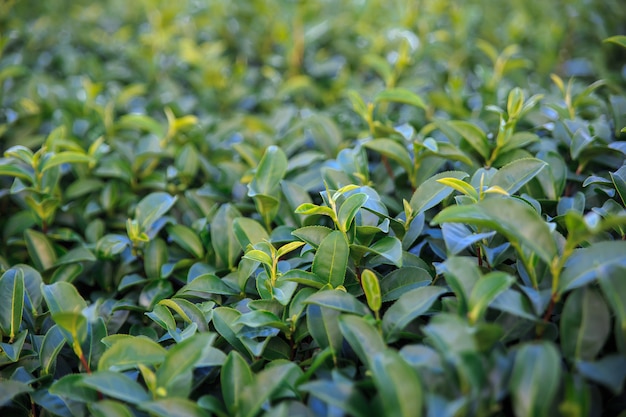In this close-up photograph taken in bright daylight, we see a dense ground cover of oblong, rectangular-shaped leaves from a single plant that fills the entire frame. The leaves vary in color from a fresh, lighter yellow-green at the top with new budding growth, to a deep, darker green towards the bottom, indicative of their age. Each leaf showcases yellow or light green veins that add to the intricate detail of the foliage. The plant also exhibits a subtle textural transition, with rough, slightly zigzag edges becoming smoother near the yellow-tinted tips. The background becomes blurrier, emphasizing the plant's depth and the overlapping nature of the leaves, some of which reflect the sunlight, enhancing the plant's vibrant greenery. The brown stems peek through, supporting this lush, detailed carpet of leaves.